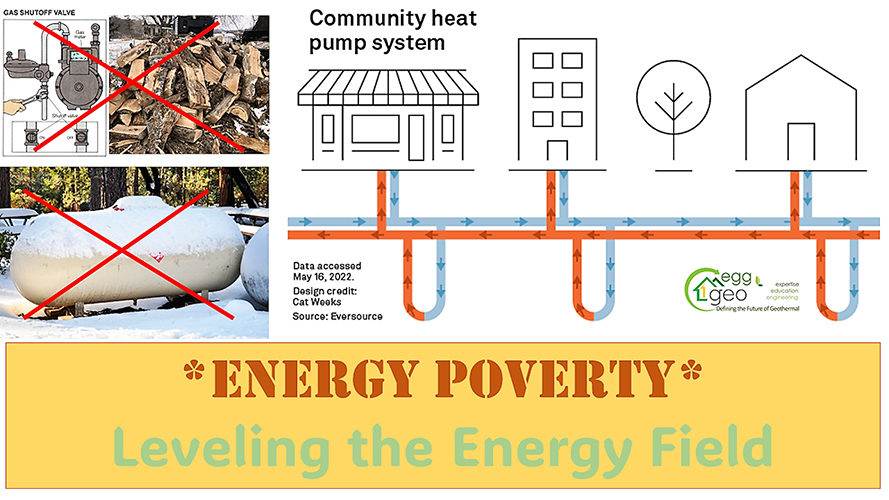This infographic features a detailed layout highlighting various elements related to energy systems and energy poverty. Dominating the bottom is a yellow banner with the message "Energy Poverty: Leveling the Energy Field." On the left-hand side, there are three distinct images: a photograph of chopped wood for a fireplace, a drawing of a gas shutoff valve, and a photograph of a snow-covered tank, possibly a propane tank. Each of these images is marked with a red X, indicating they are not preferred energy sources. 

To the right, the main focus is a simplistic line-art diagram titled "Community Heat Pump System." This diagram includes a house, a building, and a storefront interconnected by red and blue pipes, showing the flow of hot and cold air to and from these structures. Arrows in the diagram illustrate the energy exchange within the community system. Additional small text notes that data was accessed on May 16th, 2022, with design credits to Cat Week and source attribution to Eversource. The logo for Egg Geo is also present, adding to the professional context of the infographic.